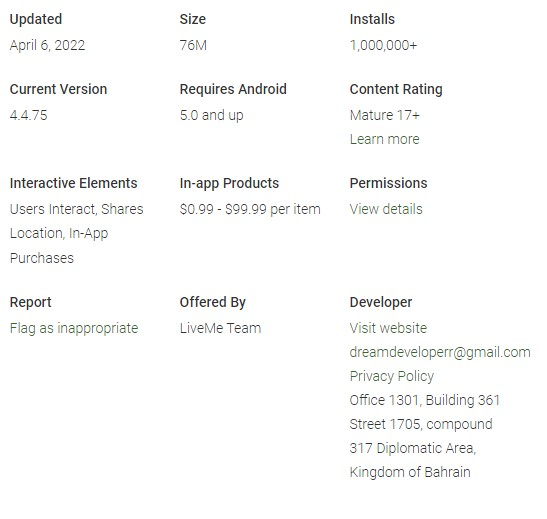The image features a detailed description of an app update on a white background. At the top left, the bold header "Update" is displayed, followed by the date "April 6, 2022" in finer text underneath. 

Below that, the category "Size" appears in bold with the capitalized first letter, stating "76M" in finer text underneath. On the right side, the bold heading "Installs" shows "1 Million+" in finer text with a plus sign.

The next line features "Current Version" in older text, marked as "4.475", followed by "Requires Android 5.0 and up" in plain text.

The "Content Rating" is labeled as "Mature 17+" with a plus sign, along with a "Learn More" link.

The "Interactive Elements" section details user interactions, sharing of location, and in-app purchases, ranging from $0.99 to $99.99 per item.

At the bottom, permissions, view details, report flag as inappropriate, and the information "Offered by Live Meeting Developer" are provided, along with options to "Visit Website" and "Privacy Policy". The address information follows.